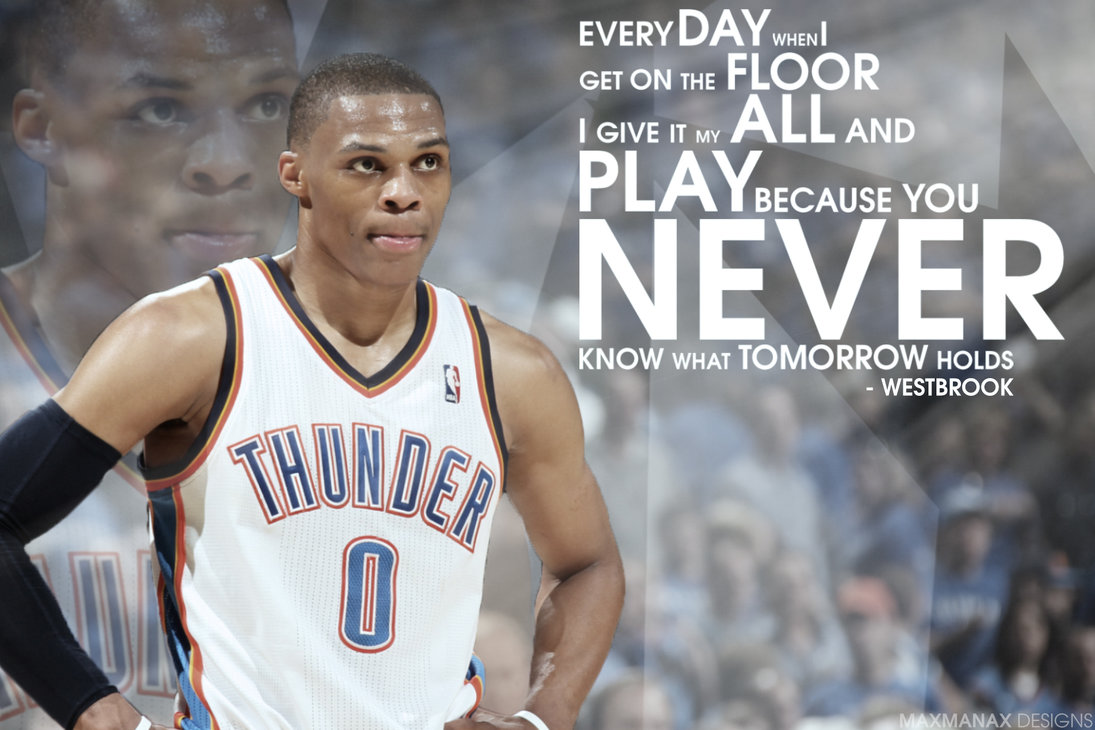The digitally generated image features a basketball player from the Oklahoma City Thunder, wearing a white sleeveless jersey with blue text and orange outlines that reads "Thunder," alongside the number zero. The player, identified as Russell Westbrook, is an African American man with a clean-shaven head, shown standing with both hands on his waist and looking upwards. He is also wearing a black elbow sleeve on his right arm and two white wristbands. In the background, there is a faded, larger shadow image of Westbrook's face, along with a blurred audience and indistinct logos. The right side of the image displays a quote in white block letters, saying, "Every day when I get on the floor, I give it my all and play because you never know what tomorrow holds," attributed to Westbrook, with "never" emphasized in larger text. The bottom right corner bears the watermark "Max Men Next Designs."